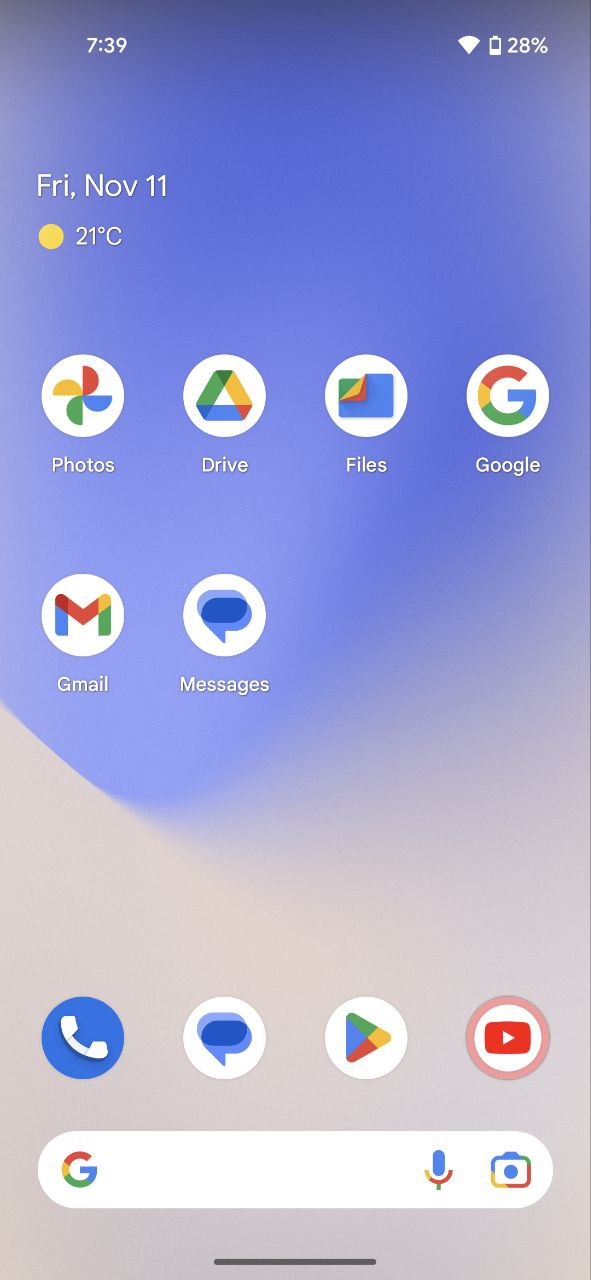The image depicts the homepage of a smartphone. The wallpaper transitions from a dark blue at the top to a lighter blue halfway down, then shifts abruptly to a grayish-pink hue towards the bottom. At the top left corner, white text displays the time as 7:39 AM. To the right, the status bar shows the Wi-Fi symbol and a battery icon indicating 28% battery life. Directly below, the white text reads "Friday, November 11th." Beneath that, a sun icon signifies clear weather with a temperature of 21 degrees Celsius.

The main screen is organized with four rows of app icons, each containing four icons per row. From left to right, the first row includes Photos, Drive, Files, and Google. The second row features Gmail and Messages. Below these, the familiar icons for phone calls, text messaging, Google Play Store, and YouTube are neatly aligned. At the bottom of the screen, a Google search bar concludes the layout, offering a convenient tool for quick searches.